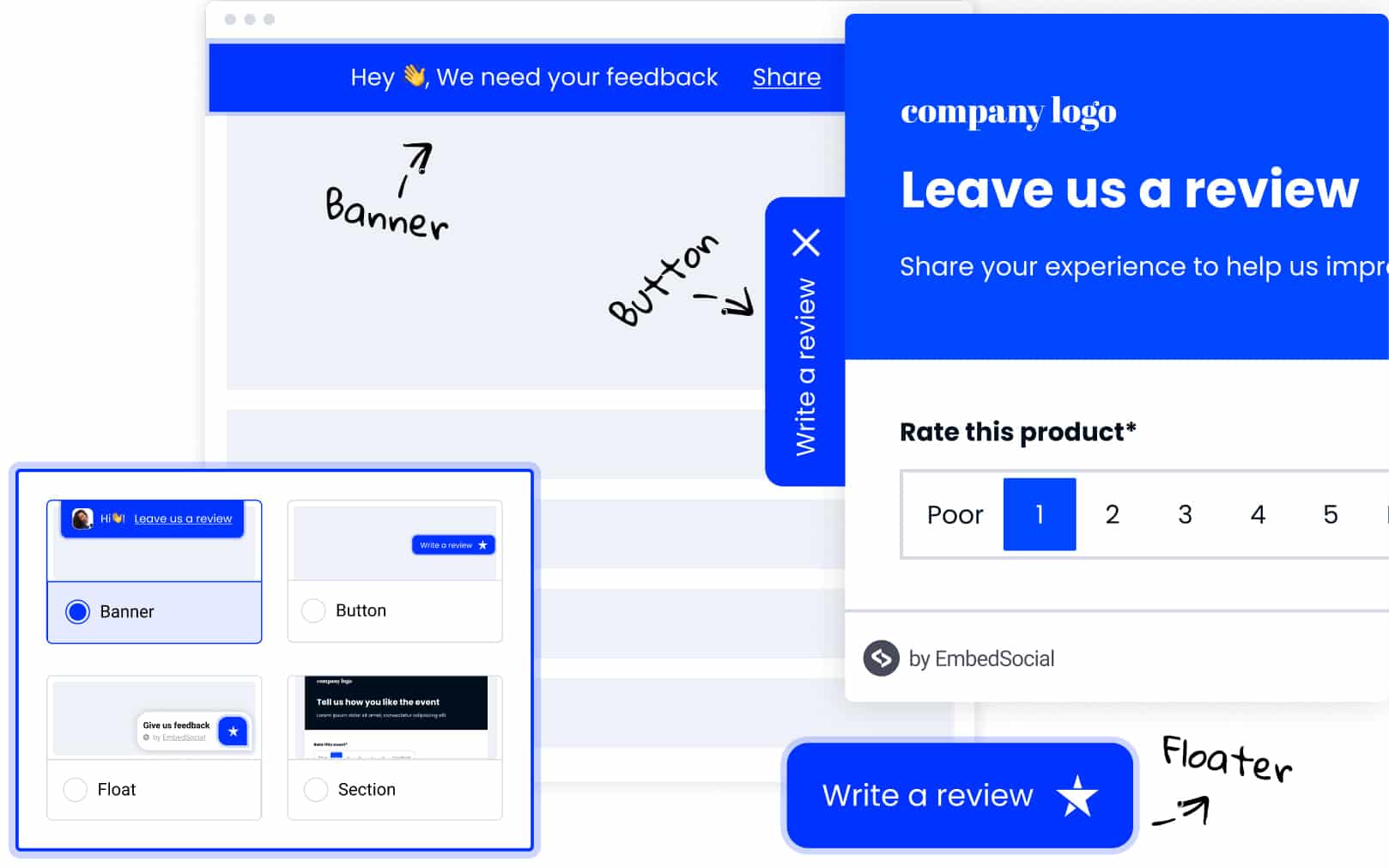This series of screenshots appears to be a detailed mock-up for a website's feedback and review interface. The collection of images seems to be an initial design phase, illustrating various elements and user interactions. 

The first screenshot captures a basic website layout with minimalistic, placeholder content. At the top, there's a royal blue banner with white text that reads, "Hey, we need your feedback." Accompanying the text is a waving hand emoji, adding a friendly touch. A hand-drawn arrow labeled "banner" points directly to this section, emphasizing its importance. Adjacent to this is another tab labeled "Write a Review," with text oriented horizontally. An X mark is positioned at the top-right corner of this blue rectangle, denoted as "button" by an arrow and text annotation.

To the right of this primary layout, there’s an additional screenshot showcasing a more detailed review page. This section features a prominent blue banner that states, "Company logo," and "Leave us a review, share your experience to improve." Below this, bold text prompts users to "Rate this product." A rectangular scale beneath this prompt ranges from "Poor" to a partially visible higher value, presumably extending the rating options up to 5. 

In the bottom left-hand corner of this segment, there's an icon indicating "by Embed Social." Directly below this, another blue "Write a Review" button is visible, marked by an arrow labeled "floater." This button is accompanied by a star symbol, signifying its function.

Additionally, a collection of thumbnail screenshots is found in the bottom left-hand corner of the overall image. These thumbnails display various configurations and options for elements like banners, buttons, and floating sections, providing a comprehensive overview of the potential design choices available for the website.

Overall, this detailed mock-up provides a polished and user-friendly interface for gathering customer feedback and reviews, ensuring an intuitive and engaging experience.